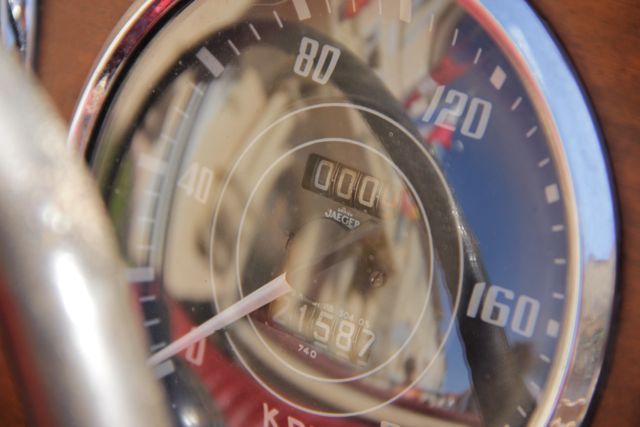The image displays a detailed view of an odometer. The odometer increments are denoted at intervals of 40, with readings at 0, 40, 80, 120, and 160. At the center of the display, the brand name "Jaeger" is prominently featured, along with the mileage reading "21,587 miles." The odometer's outline is sleek and silver, with a reflective surface that catches the light. The background of the image is a warm, light brown, providing a subtle contrast to the silver outline. In the lower left corner, part of a silver steering wheel is visible, adding to the automotive context of the image.